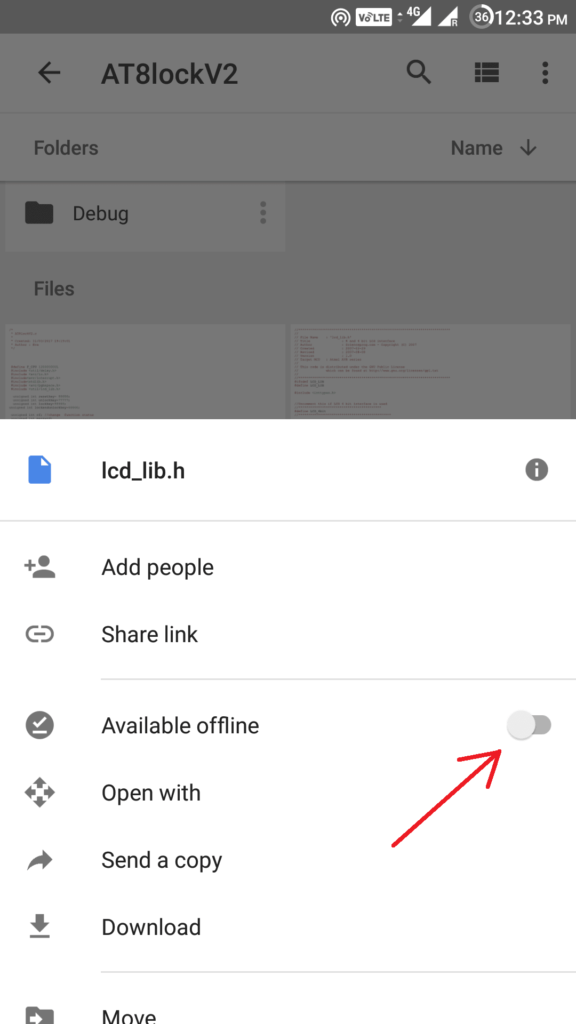The image depicts a smartphone screen displaying the "AT8 Lock V2" interface. In the top left corner, there is a back arrow. Nearby, icons for a magnifying glass and settings can be seen, indicating search and configuration options respectively. Just above this section, the status bar shows a hotspot connection, 4G and VoLTE signals, the battery level at 36%, and the current time of 12:33 PM.

Underneath the "AT8 Lock V2" label, a folder icon is present on the left-hand side, and on the right, there is a dropdown arrow next to a name. Further down, the interface displays a gray box containing a folder icon labeled "Debug" and an ellipsis (three dots), which likely lead to more settings options. Below this, there are the words "Files" and partial display of two documents with minuscule text.

Beneath the gray box, on a white background, sits a blue folder icon labeled "lcdlib.h." Adjacent to this, there are options to add people, share a link, and toggle the file's offline availability, which appears to be enabled. To the left of these options, there is a diagonal red arrow pointing upwards. Additional action buttons including "Open with," "Send a copy," "Download," and "Move" are displayed, each accompanied by their respective icons.